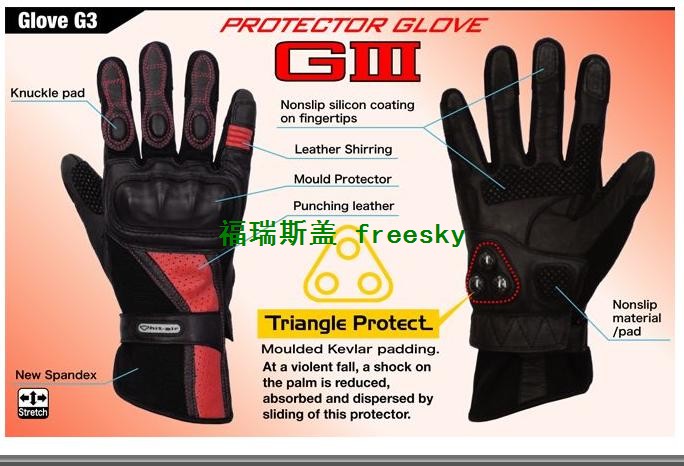The photograph features an advertisement for Protector Glove G3, showcasing a pair of industrial-style or motorcycle-type black leather gloves. The background transitions from a deep red at the corners to a lighter shade in the middle, with a small black section in the top left corner displaying "GLOVE G3" in white letters. The centerpiece text, also in red, prominently states "PROTECTOR GLOVE G3," accompanied by descriptive labels.

On the left-hand side, the image illustrates the back of the glove, highlighted by striking red lines that outline the finger joints and a long red stripe extending down its right side. A black strap adorned with a silver image encircles the base of the glove. In contrast, the right-hand side of the image reveals the palm of the glove, which appears textured and features a triangular-shaped Velcro closure.

Several arrows point to various features, each accompanied by text that details the glove’s sophisticated protective elements. These include knuckle pads, non-slip silicone coating on the fingertips, leather shirring, mold protector, and punching leather. Significantly, the glove highlights its "Triangle Protect" feature, symbolized by a triangular emblem with three small circles, denoting molded Kevlar padding designed to mitigate impacts. The advertisement explains that in the event of a violent fall, the gloves are engineered to reduce, absorb, and disperse shock through this advanced padding system.

Complemented by a mix of English text and Asian font, the advertisement meticulously diagrams the gloves’ offerings, illustrating both the aesthetic and functional attributes that make them ideal for laborious tasks or motorcycling. The visual depiction, combined with thorough annotations, effectively conveys the gloves' durability and comprehensive protection.